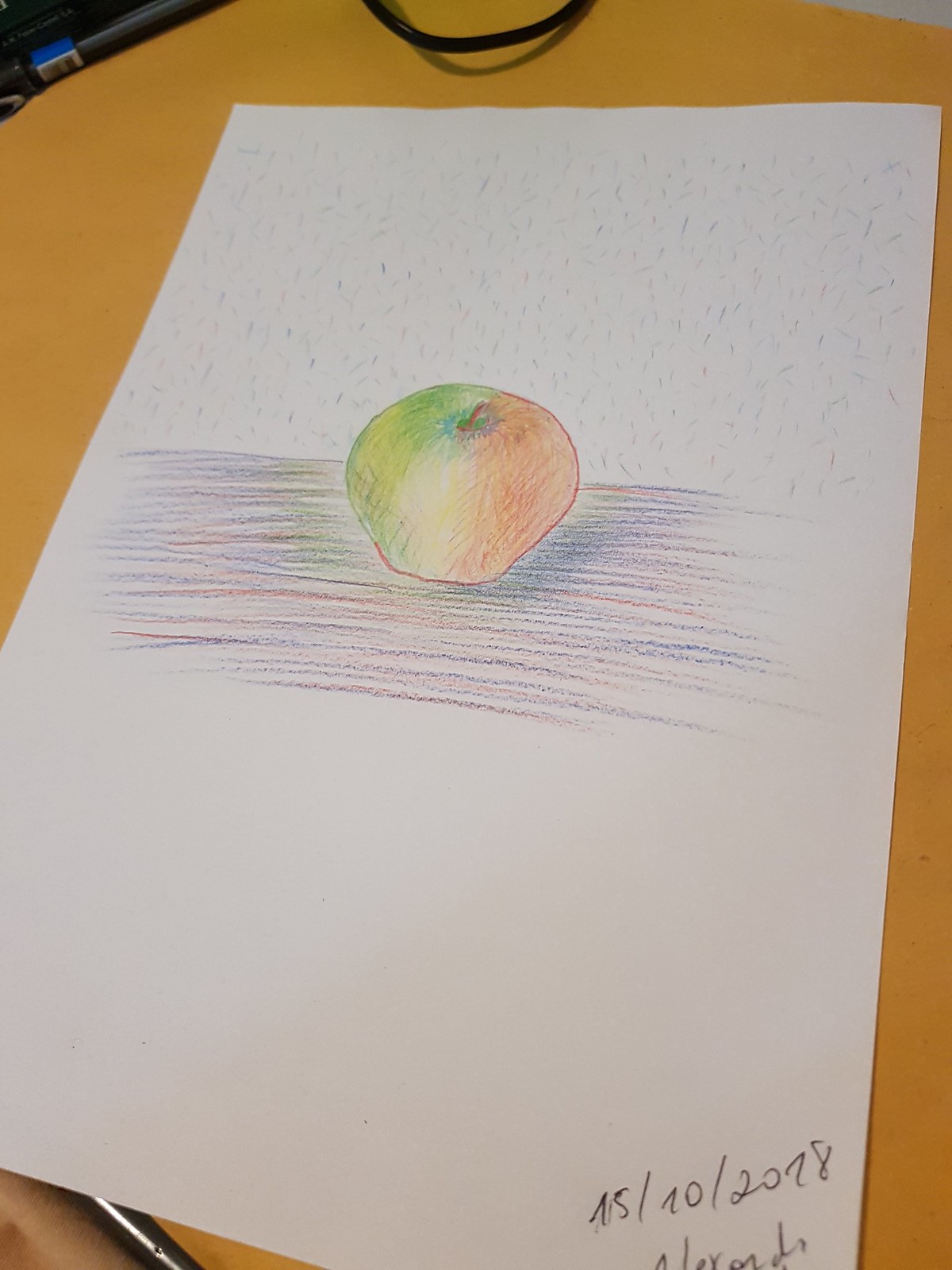The photograph depicts a detailed colored pencil drawing on a white rectangular sheet of paper, oriented vertically on a yellowish-orange desk. In the upper left corner of the desk, parts of a black cord and another black object are visible. The drawing, occupying the upper two-thirds of the page, features a realistic apple shaded with multiple colors: green on the left, red on the right, and interspersed with hints of gold, pale yellow, and brown. An interesting choice of colors and shading gives the apple a vibrant, almost psychedelic quality. Below the apple, horizontal hatching in shades of red, purple, and blue suggests a table surface. Above this, light gray speckling indicates a backdrop. The lower third of the page is blank, except for a signature and the date "15-10-2018" in the lower right corner.